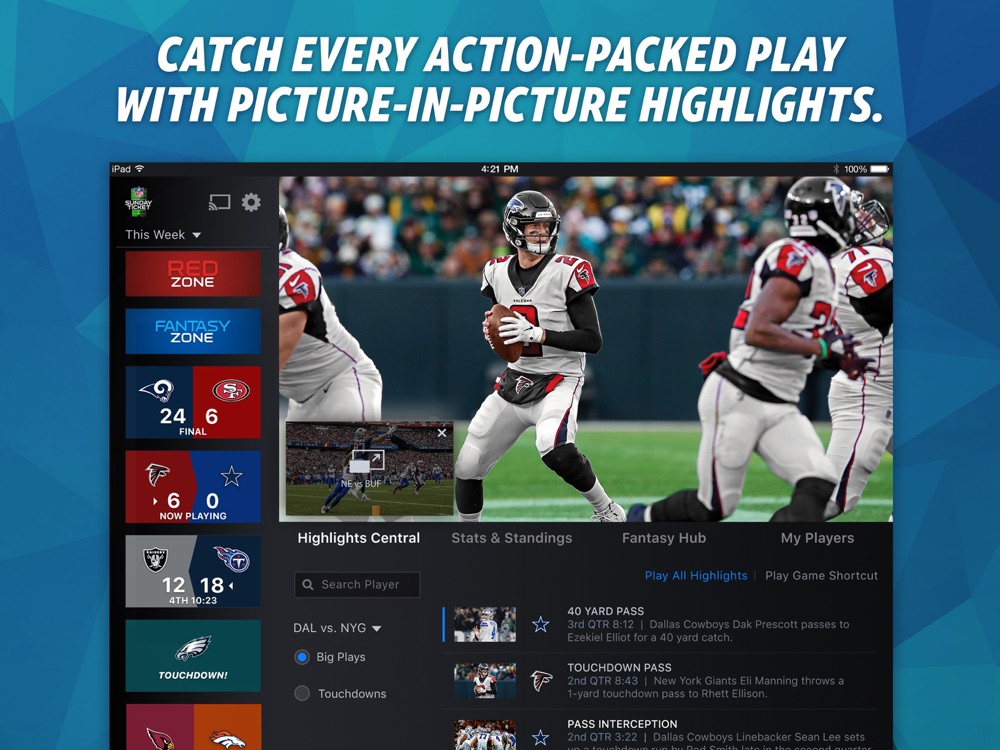This image is an advertisement-like poster promoting a sports streaming app designed for an iPad. The central focus is on a live football game featuring Matt Ryan playing for the Falcons, captured mid-action as he prepares to throw a pass. In the lower left corner, a smaller picture-in-picture window displays another game, likely involving the Detroit Lions, illustrating a wide receiver catching the ball. Surrounding the main screen, a menu interface offers various features such as highlights, central stats, standings, Fantasy Hub, and My Players. The left sidebar lists different ongoing games, including matchups like Rams vs. Niners and Falcons vs. Cowboys. The app appears to be a comprehensive hub for sports enthusiasts, providing easy access to live games, highlights, and intricate details about ongoing matches, all on an iPad platform.